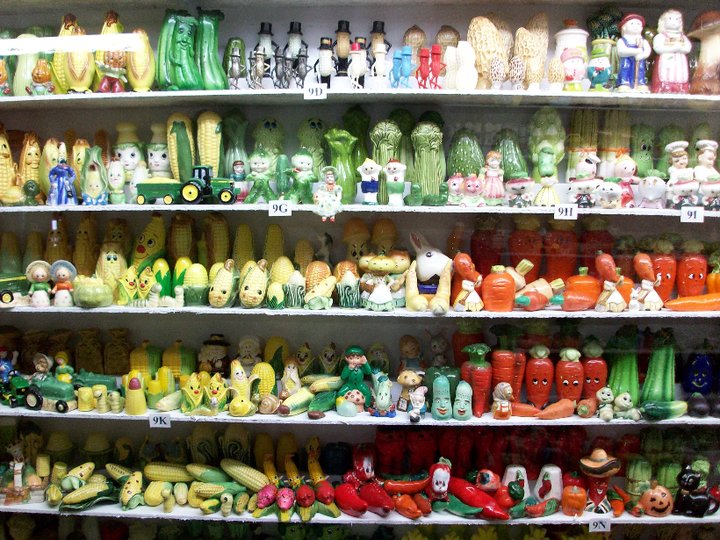The image is a vibrant photograph depicting six shelves brimming with an eclectic collection of ceramic objects. The shelves are filled with predominantly food-shaped novelty items, many of which are salt and pepper shakers. Ears of corn, chili peppers, carrots, cucumbers, squash, zucchini, and celery are all represented, with several featuring whimsical faces and eyes, creating a delightful array of anthropomorphized produce. The collection is highly colorful, with yellow from the corn, red from the chili peppers, and green from the various squashes standing out. Amongst the vegetables, there are also humanoid figurines, including multiple Mr. Peanut items, as well as small figures of boys and girls styled in a vintage mid-20th-century aesthetic. The display, likely a collector's treasure trove, captures a sense of nostalgic charm and playful artistry, evoking a country scene of smiling, characterful vegetables.